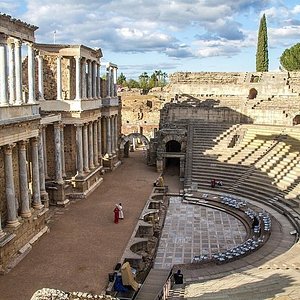The image captures an ancient amphitheater reminiscent of Greek or Roman architecture, with a backdrop of deteriorating historic ruins. The amphitheater features stone-carved seating that descends step by step to a sunken, semi-circular stage paved with large red bricks. Flanking the amphitheater are buildings adorned with white marble columns, though some appear decrepit. A sizeable shadow, presumably cast by an unseen adjacent building, blankets part of the ruins and trees in the background. Two tourists are walking past the amphitheater, adding a small touch of life to the otherwise somber scene under a partially cloudy sky. A tall, slender tree is visible in the upper right of the image, juxtaposing the human-made structures.